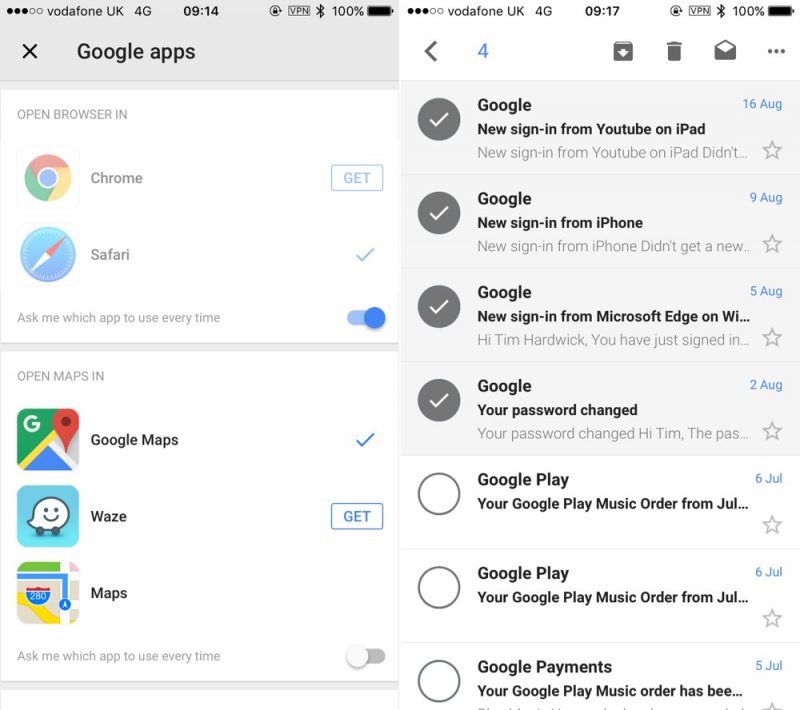**Descriptive Caption:**

The image comprises two iPhone screenshots, showcasing various app settings and notifications. 

**Left Screenshot:**
- **Top Status Bar:**
  - Signal: 3 out of 5 dots
  - Carrier: Vodafone UK
  - Network: 4G
  - Time: 9:14 AM
  - Icons: Lock, VPN, Bluetooth, and 100% battery indication
  
- **Content:**
  - Google Apps: An 'X' to exit
  - **Browser Preferences:**
    - **Chrome:**
      - Background: White
      - Logo: Chrome logo
      - Button: Blue "Get" button
    - **Safari:**
      - Logo: Safari logo
      - Status: Blue check mark indicating selection
  - **Choice Prompt:**
    - Label: "Ask me which app to use every time"
    - Control: Slider activated to the right
  - **Map Preferences:**
    - Label: "Open maps in"
    - **Google Maps:**
      - Logo: Google Maps logo
      - Status: Check mark indicating selection
    - **Waze:**
      - Logo: Waze logo
      - Button: Blue "Get" button
    - **Apple Maps:**
      - Logo: Apple Maps logo
    - **Choice Prompt:**
      - Label: "Ask me which app to use every time"

**Right Screenshot:**
- **Menu Bar at Top:**
  - Indicators: Left arrow, number 4 (in blue), down arrow in a box, trash can, envelope, and three dots for more options
  
- **Content:**
  - **Notifications:**
    - **Google Alerts:**
      - "New sign in from YouTube on iPad, August 16th"
      - "New sign in from iPhone, August 9th"
      - "New sign in from Microsoft Edge on Windows (WI), August 5th" (addressed to Tim Harwood)
      - "Your password change, August 2nd"
      - "Your Google Play music order from July 6th" (repeated twice)
      - "Your Google Payments order, July 5th"

This comprehensive display shows a juxtaposition of app settings and email notifications, providing detailed visibility into the user's preferences and recent account activities.